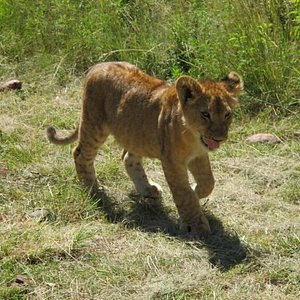In this photograph, a young lion, likely a juvenile male or small female, is captured in mid-stride as it walks along a grassy terrain. The vibrant mixture of orange, gold, and brown on its fur, with darker patches accentuating its legs and tail, highlights its alert and healthy disposition. The lion's tail droops low but perks up at the end, adding a dynamic curve to its posture, mirrored by the bent left front paw as it takes a step. The setting is lush, with a combination of short, well-trodden grass underfoot and taller, greener grass surrounding it, sprinkled with small gray stones. The lion's mouth is open with its tongue hanging out, and its ears are perked up, conveying a sense of curiosity and vitality. A faint shadow of the lion on the grass adds depth to the image, suggesting a bright, sunny day in a possibly warm climate.